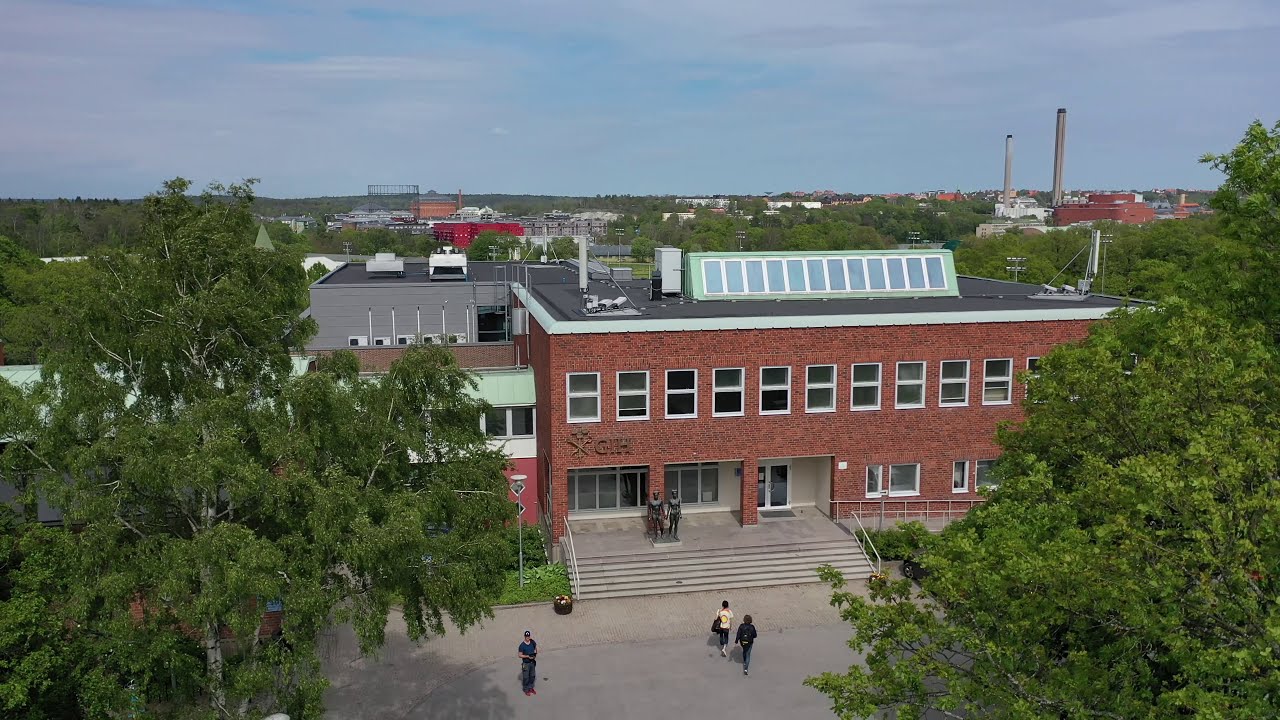The image captures a red brick building adorned with numerous windows, hinting at it potentially being a school or an institutional facility. In front of the building's steps, several people are walking towards it, many carrying backpacks, suggesting a campus-like setting. A man, distinguished by his red shoes, black cargo pants, blue t-shirt, and black hat, stands prominently to the left of the entrance, seemingly engaging with a drone camera as he holds a device. The facade of the building displays the letters "GH" alongside a peculiar cross symbol topped with a Mickey Mouse head. Overhead, a clear blue sky with light clouds forms the backdrop. Partially obstructing the view are trees, stretching across the image from left to right. Beyond the main building, a cityscape unfolds, featuring similar structures, large exhaust pipes from factories, and an array of green trees interspersed among the urban features, depicting a mid-sized Midwestern city without towering skyscrapers.